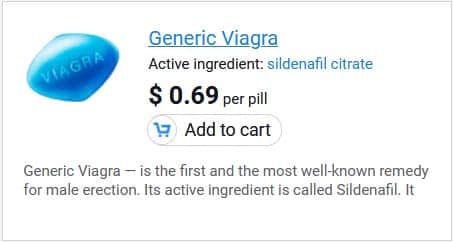The image is a rectangular advertisement, approximately 50% wider than it is tall, featuring a promotional message for Viagra. The focal point of the image is a large, white box with a thin gray outline, positioned centrally. In the upper left corner of the box, there's a blue Viagra pill, which takes up about 25% of the image's height and width. The pill is oriented diagonally, tilted to approximately a 230-degree angle. The word "Viagra" is inscribed on the pill, following the same diagonal direction.

To the right of the pill, centrally aligned, the text "Generic Viagra" appears in light blue with an underline. Beneath this, the phrase "Active Ingredient:" is written in black, followed by "sildenafil citrate" in blue. Further down, the text "69 cents per pill" is prominently displayed in bold black font, larger than the preceding text. Below this, there is a button featuring a shopping cart icon on the left, with the words "Add to Cart" in black.

At the bottom of the image, there are two lines of left-aligned text, written in a smaller black font. The text reads: "Generic Viagra - is the first and most well-known remedy for male erection. It's active ingredient is called sildenafil it," though it is incomplete and trails off abruptly.